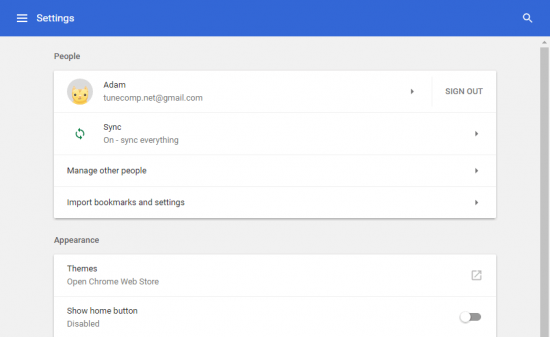**Settings Page of a Web Browser - Comprehensive Overview**

At the top 10% of the page, a vivid blue bar spans the width, contrasting sharply with the rest of the layout. On the left side of this bar, three horizontal lines are followed by the word "Settings," indicating the section of the browser currently being viewed. Towards the right corner of this blue section, a white search icon is prominently displayed.

Below the blue header, the background transitions to a gray tone, overlayed with two distinct white boxes, each demarcated by thin lines. The first white section pertains to "People." Here, a large area contains the user's avatar, an image of a yellow cat. To the right of the avatar, the name "Adam" is displayed, beneath which the email address "tooncomp.net@gmail.com" is listed. On the far right side of this section, there is a right-facing arrow, and beside it, a "Sign out" button provides an option for the user to log out.

Directly beneath this segment, the words "Sync" appear, indicating the synchronization status. It states "On - sync everything" with a sync button positioned to the left. Following this, two sections labeled "Manage other people" and "Import bookmarks and settings" are listed, each accompanied by a right-facing arrow on the far right.

Further down, the section titled "Appearance" begins. Within the white box under this heading, users can click on "Themes," which directs them to the "Open Chrome Web Store." To the right of these options, a clickable icon is present. Additionally, there is an option to "Show home button," which is currently disabled but can be activated via a toggle switch located to the right of the text.